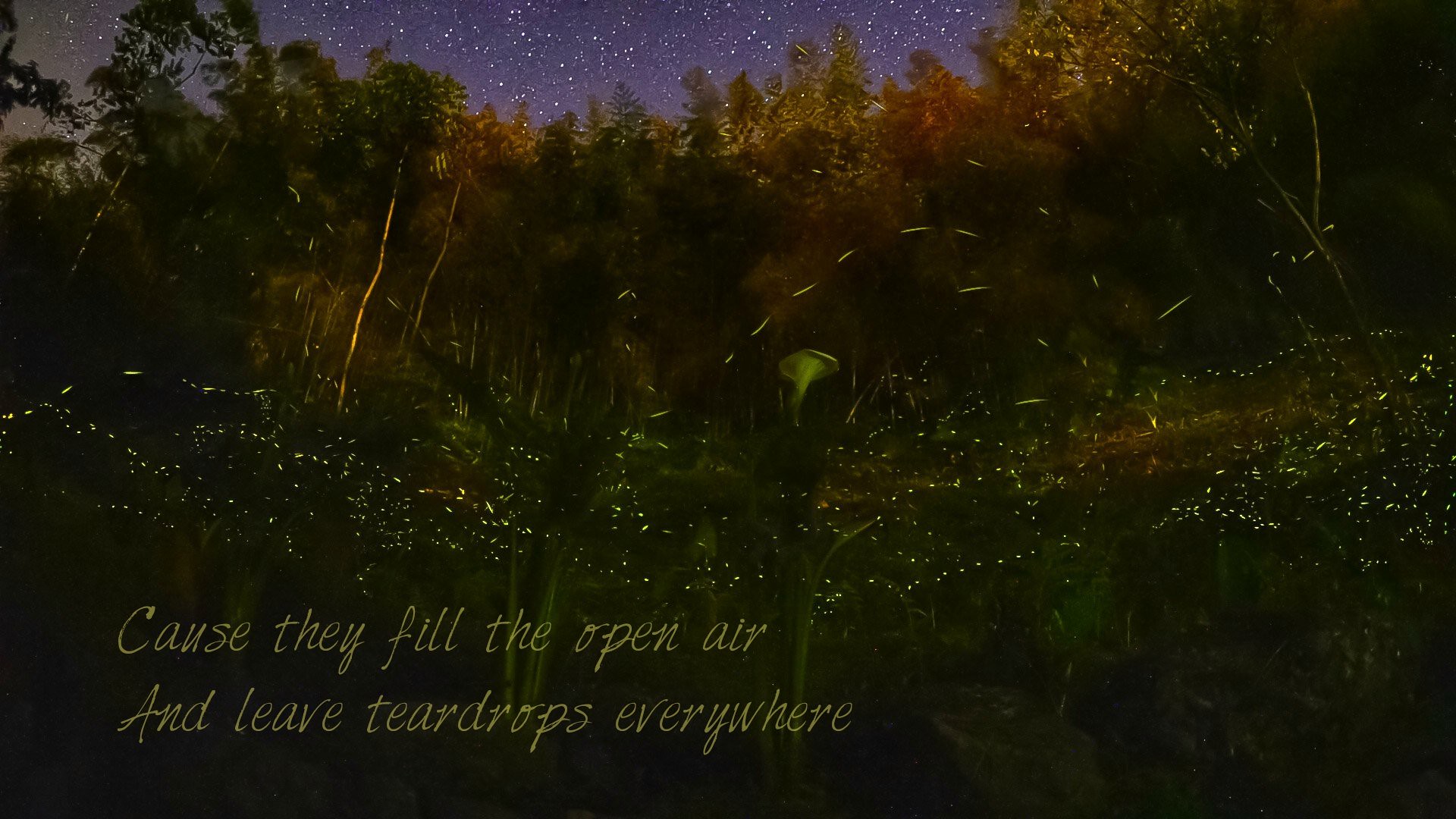This image captures a dark, enigmatic scene dominated by deep black and brown hues. At the top, a star-studded night sky casts a faint light on the very tips of the silhouetted trees, creating a serene yet mysterious atmosphere. The foliage appears to have rusty brown tones on the right-hand side and center, gradually transitioning into the green vegetation below. In the midst of this dark greenery are some indistinguishable white specks. Near the bottom left corner of the image, written in white text, are the words, "'cause they fill the open air and leave teardrops everywhere," adding an element of intrigue to the overall composition.